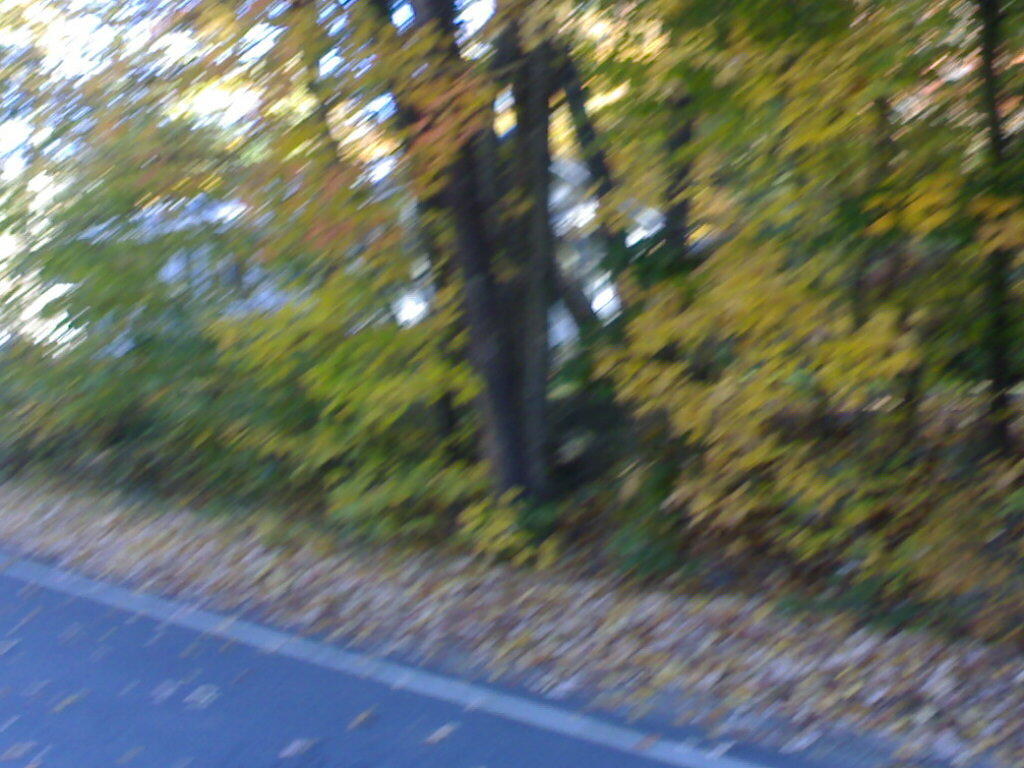The image appears to be taken from a moving car, capturing a roadside scene dominated by a dark gray road with a white line marking its edge. The lower left corner of the image showcases the road, which angles downwards to the right. Adjacent to the road, the ground is covered in a thick layer of fallen leaves, predominantly brown and yellow, indicating an autumn setting. A cluster of tall, slender trees lines the roadside, their leaves displaying a vibrant mix of yellow, green, and hints of orange that verge on red. The trees obscure the sun, casting the area in a gentle shadow, while the sky visible through the foliage appears clear. The photograph is notably blurry, suggesting it was taken mid-motion, adding a sense of dynamic imperfection to the scene.